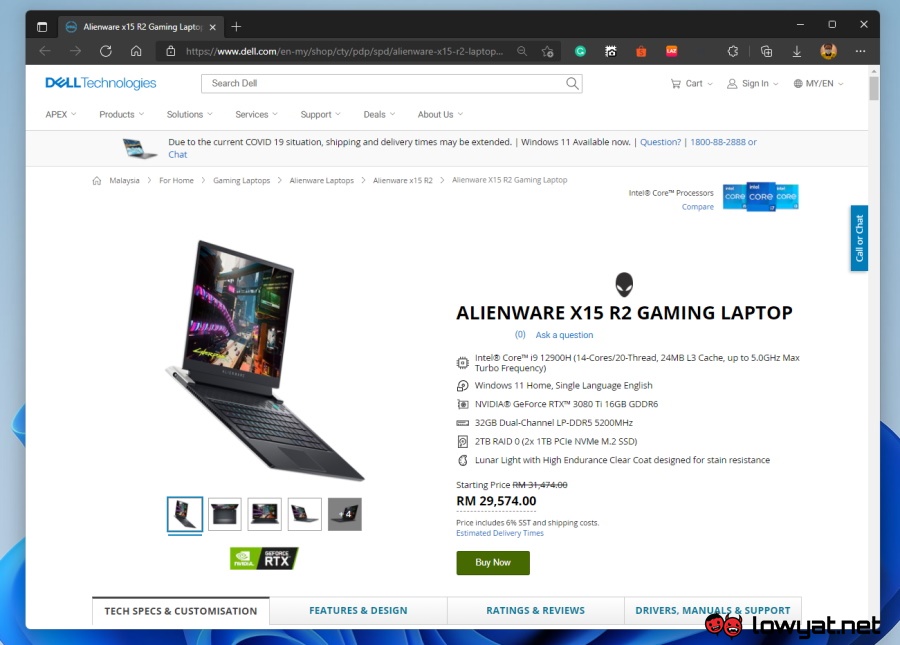A detailed description of the webpage as follows:

The webpage has a predominantly white background with a blue outline. At the bottom, the blue merges with black, and the bottom right corner is shaded gray. 

At the top left corner, the Dell Technologies logo is prominently displayed. Next to it, there's a search bar labeled "Search Dell." Below this is a gray rectangle containing a small image of a laptop. Beside the image, a notice in black text reads: "Due to the current COVID-19 situation, shopping and delivery times may be extended. Windows 11 available now."

Underneath this, the webpage includes a navigation bar with labels "Homepage," "Malaysia," "For Home," "Gaming Laptops," and "Alternative Laptops." There are additional unreadable menu items, one of which partially reads "Something Gaming Laptop."

The lower section features a larger image of a laptop, with five smaller thumbnail images below it showcasing different views of the laptop—side, top, and front angles. 

Centered on the page is the bold, black text "Alienware X15 R2 Gaming Laptop," accompanied by a small alien head icon above the "R2." Below this, specifications are listed, indicating the machine runs on Windows 11, includes 32GB of RAM, and features a 2TB RAID. The laptop's cooling technology is marketed under the term "Lunar Lite with high endurance." The price is listed as RM 29,574. There's also a green "Buy Now" button.

At the very bottom, four individual rectangles span the width of the page. The first rectangle is white, and in black text, it reads "Tech Specs and Customization." The remaining three rectangles are gray, with blue text listing "Features and Design," "Ratings and Reviews," and "Drivers, Manuals, and Support," respectively. Underneath the "Drivers, Manuals, and Support" section are small icons resembling demonic faces with sharp teeth, next to the text "LOWYAT.NET" in black letters.